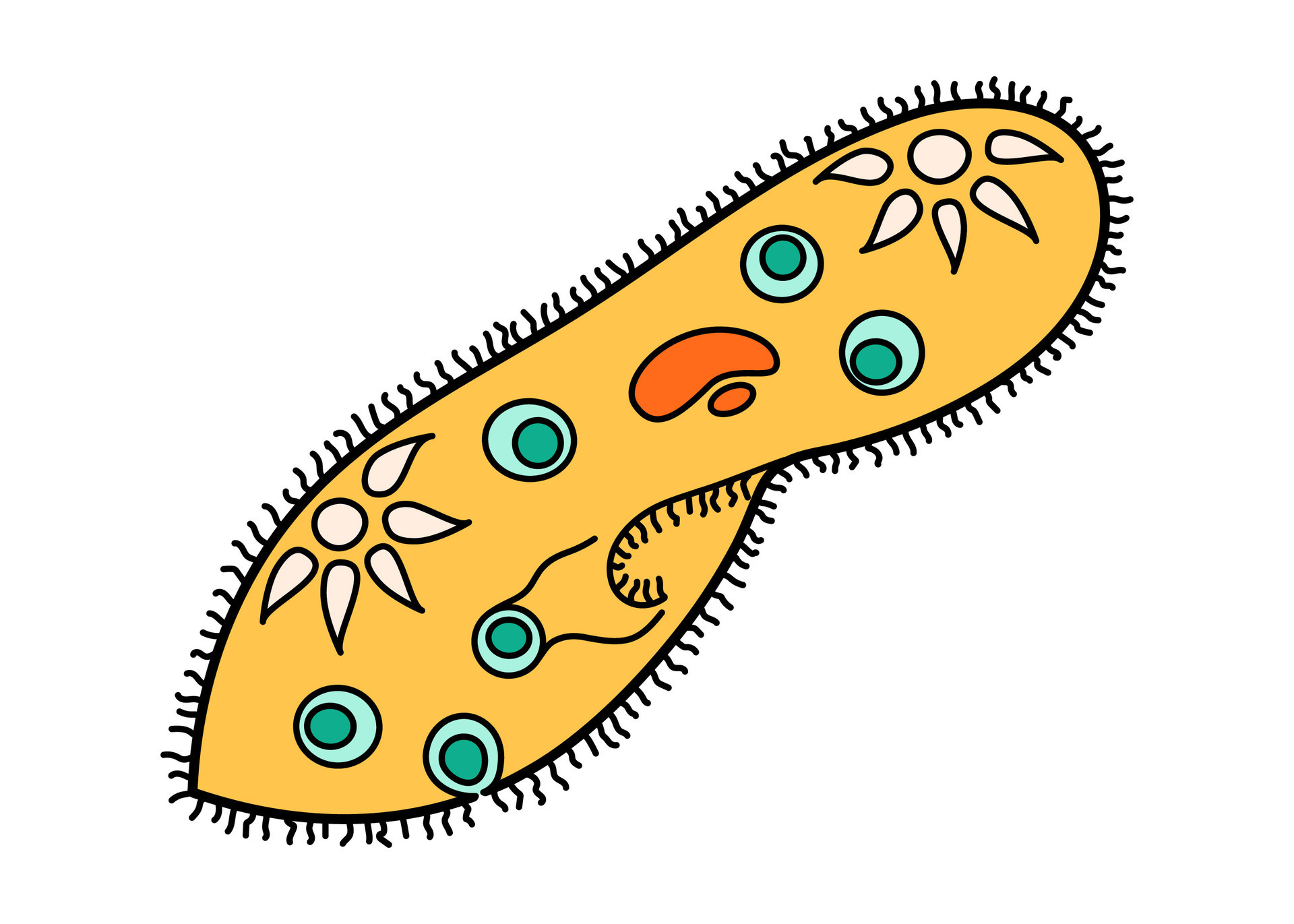This image is a detailed digital illustration of a paramecium, presented in a cartoon style to highlight various anatomical features. The paramecium is primarily colored yellow with a rounded top, angled toward the left, and outlined in black. Along the perimeter, there are numerous small black squiggly lines representing cilia, totaling approximately 200, which aid in its locomotion within a microscopic environment.

At the anterior (top right), a yellow-colored contractile vacuole is visible, mirrored by a similar posterior contractile vacuole at the bottom left. Centrally located, the micronucleus and macronucleus are depicted in shades of orange or red. Scattered throughout the paramecium are green-colored food vacuoles, resembling eye spots with darker green central parts akin to pupils. Additionally, there is a gullet, resembling an open mouth, positioned to the side.

The paramecium’s interior, or ectoplasm, is rendered in a light tan hue. This complex structure is all displayed against a white background, making the detailed components stand out vividly.